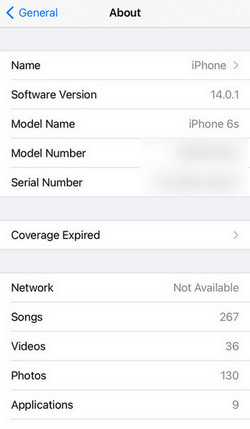A detailed and cleaned-up caption for the image described:

---
A screenshot of an iPhone screen displaying the 'About' section in the 'General' settings menu. In the upper left corner, a blue back arrow is visible, indicating a way to return to the previous menu. Next to the arrow, the word "General" is highlighted in blue. Centrally positioned at the top of the screen, the title "About" is prominently displayed in bold black letters.

Just below the title, a gray separator bar spans the width of the screen, followed by a white bar containing the label "Name" on the left and "iPhone" on the right, accompanied by a right-pointing arrow. The next row lists the "Software Version" with the value "14.0.1" on the right. Beneath that, the "Model Name" is specified as "iPhone 6S." The "Model Number" and "Serial Number" entries are present but redacted. Another gray separator bar appears below these details.

Continuing down, another white bar lists "Coverage Expired" on the left, with a right-pointing arrow on the right. Following a third gray separator bar, the next white bar shows "Network" on the left and "Not Available" on the right. Below this, there are entries for "Songs" with a count of "267," "Videos" with "36," "Photos" with "130," and "Applications" listing "9" items on the right. 

The image concisely displays essential device information and statistics within the 'About' section of an iPhone's settings.
---